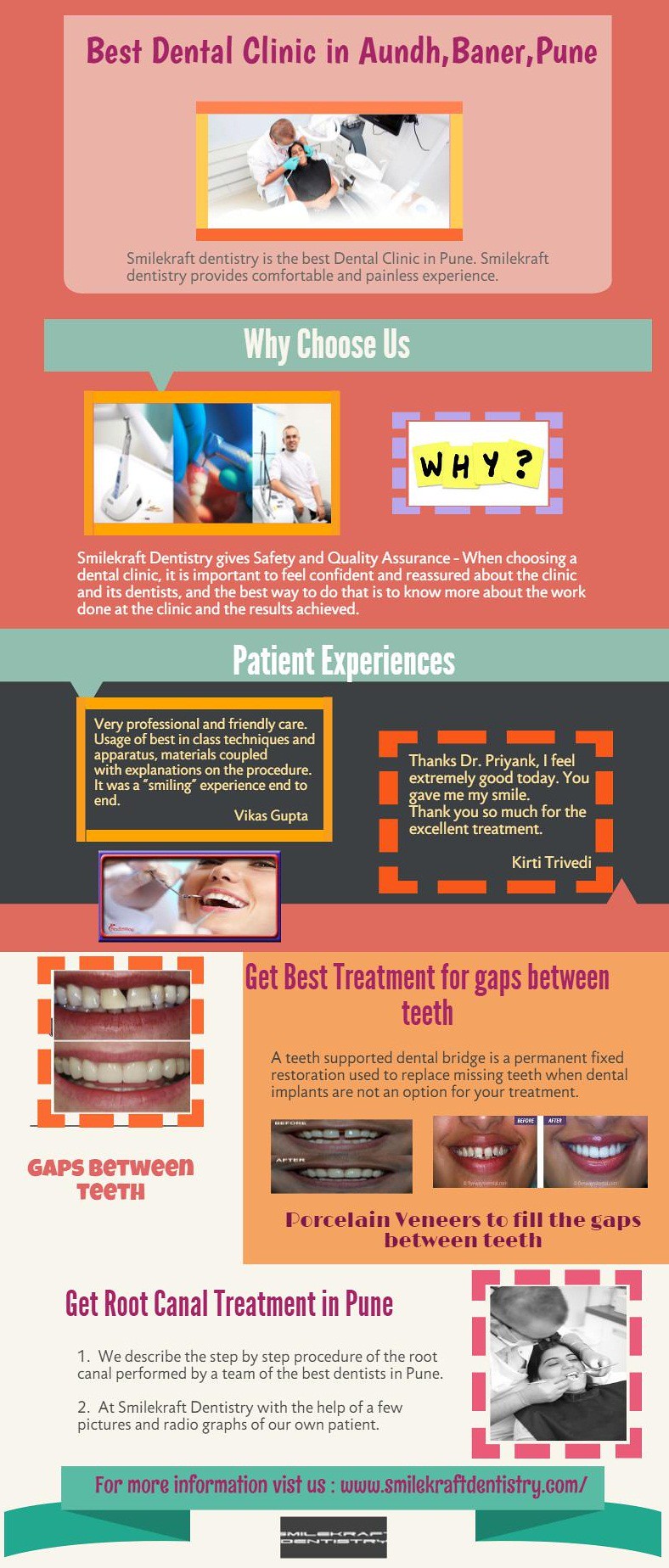The promotional flyer for Smilecraft Dentistry, displayed in various colored squares, highlights its status as the "Best Dental Clinic in Pune," specifically in Aundh and Baner. The top section features a peach-colored box with extensive text detailing the clinic's advantages—emphasizing a comfortable and painless experience, safety, quality assurance, and professional, friendly care. It underscores the importance of patient confidence by showcasing successful dental work and techniques.

Central to the design, an orange-outlined image depicts a dentist attending to a patient, with a black speech bubble stating, "Why Choose Us?" There's also a blue box with white text introducing patient experiences and testimonials. Patient stories in navy, orange-dotted, and yellow-bordered boxes affirm the clinic’s excellence.

The flyer mentions specific treatments such as gap correction, displayed with before-and-after photos under "Get Best Treatment for Gaps Between Teeth," and root canal treatments. The lower section features a tan box with pink lettering and a summary paragraph. Finally, a blue banner at the bottom directs viewers to the clinic's website for further information, ensuring comprehensive visibility of their offerings.